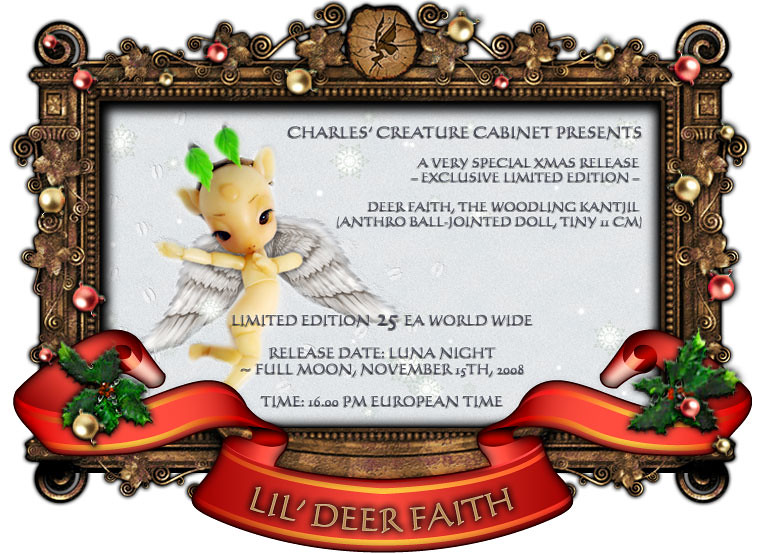This is a detailed, wide rectangular digital event invitation, creatively designed with an intricate brown wooden frame adorned with numerous floral patterns interwoven with curved vines, shiny red and gold bulbs, Christmas bells, and trees. On the sides of the frame are circular designs encompassing a winged woman in flight. The main background of the invitation is white, featuring a character on the left resembling a beige reindeer or fairy with yellowish tones, white wings, and green leaves on its head. The character also sports subtle, black eyes giving it an enigmatic appearance. Below this scene is a striking red ribbon trimmed with golden lines, displaying the words "Lil Deere Faith" in gold font. To the right of the character, the text reads: "Charles Creature Cabinet Presents a Very Special Xmas Release Exclusive Limited Edition." Additional event details and a festive theme further accentuate the announcement, promoting a limited release worldwide, set for a significant date under a full moon on November 15, 2008, at 16:00 PM European time, enhancing the sense of exclusivity and celebration.